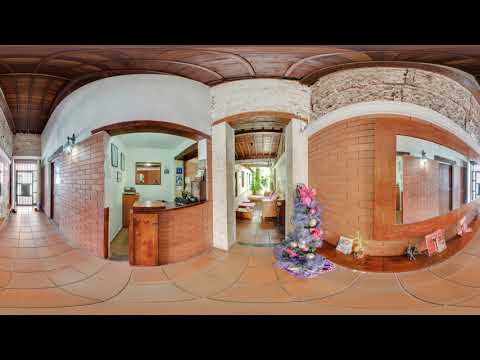The image depicts a highly detailed, possibly computer-generated panoramic view of what could be a grand, interior space, reminiscent of a cathedral or a high-end mall and imbued with an intricate blend of architectural styles. Dominated by a warm color palette of peach, brown, and orange, the floor and walls are primarily composed of orange brick, while the ceiling features dark brown paneling. 

In the central area, a multitude of colorful, spring-like flowers in shades of pink, purple, and blue are prominently displayed, contributing to the vibrant atmosphere. The right side showcases closed rooms and a gated entrance, while the left side presents a hallway leading to another part of the structure, possibly extending into a passage near a kitchen decorated with white walls and wooden cabinets. Off-center, the lounge area is furnished with chairs and tables, adding to the sense of a well-used space.

The presence of elaborate arches and marble stone details in gray and beige further augment the ornate aesthetic, echoing the feeling of a high-end or religious venue. The overall impression conveys a complex, opulent environment that merges traditional and modern elements, possibly altered or viewed through a panoramic lens that introduces certain visual distortions.